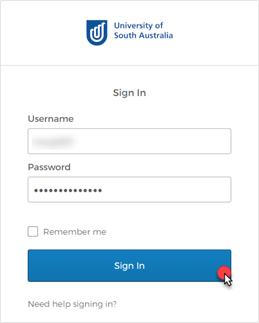The image is a detailed screenshot taken from an online application web page for the University of South Australia. The content is presented within a vertically oriented, rectangular framed window with a clean, white background. 

At the top left corner of the window is the university's blue logo, which is styled as a bold, U-shaped figure interspersed with smaller white U shapes within it. To the right of the logo, the text "University of South Australia" is written in a matching blue color. 

Directly beneath this header, the word "Sign in" is displayed in grey. 

Below the "Sign in" text, there is a text box for the username, with the label "Username" in grey positioned to the left of the text box. 

Following this is another text box designed for password entry, identifiable by the small black dots that obscure the text. The "Password" label appears in grey above and to the left of this box. 

Further down, there is an empty check box accompanied by the text "Remember me" to its right. 

Finally, at the bottom of the form is a prominent blue button labeled "Sign in." 

This screenshot effectively captures the essential elements required for user login on the university's online application page.